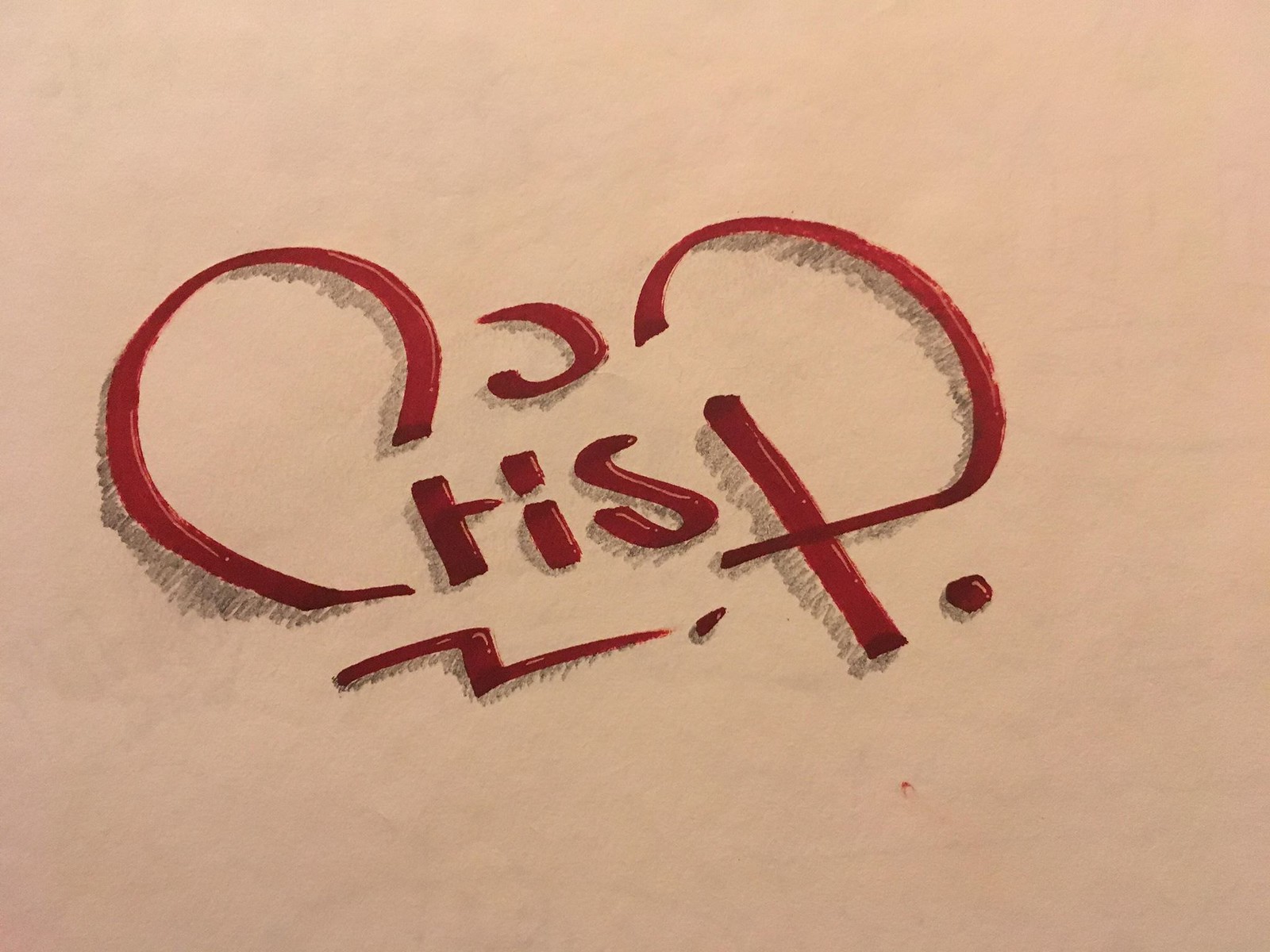The image displays an ornate drawing featuring the word "crisp" rendered in red letters against a pink background. The lettering style includes a large, elegantly curved "C," followed by a smaller "r" and "i." The "i" is adorned with a simple period topped by a decorative circle. Continuing the word, a small "s" precedes a prominently large and curved "P." Additional artistic elements include a couple of dots placed below the lettering, enhancing the word's stylized appearance. Each letter is further accentuated with subtle shadowing, adding depth and an intriguing visual effect to the design.